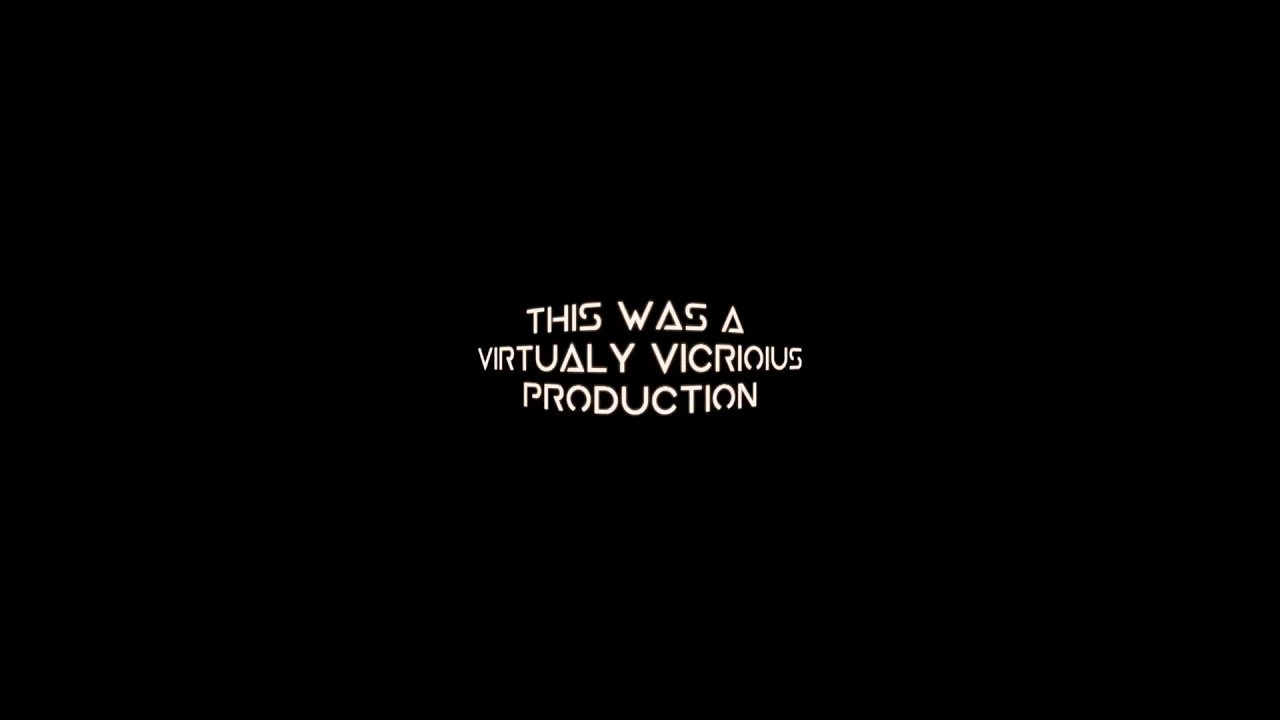In this image, we see a solid black rectangular background that takes up the entire frame. Centered against this backdrop is white text in a thin, all-caps font. The text is arranged in three lines, each line center-justified both horizontally and vertically within the black rectangle. The white text stands out clearly against the black background, and there is no other content in the image, leaving a lot of empty space. The lines of text appear to have a slight 3D effect, as if bending towards the viewer, creating a subtle illusion that enhances the visual appeal. The text reads: 

- "THIS WAS A"
- "VIRTUALLY VICARIOUS"
- "PRO-DUCK-TION"

Additionally, the straight-lined letters like A, L, and H are very precise, while the A's resemble triangles with a small portion of the bottom left corner missing. The overall impression is minimalist and modern, resembling something you might find in online digital media or clip art.